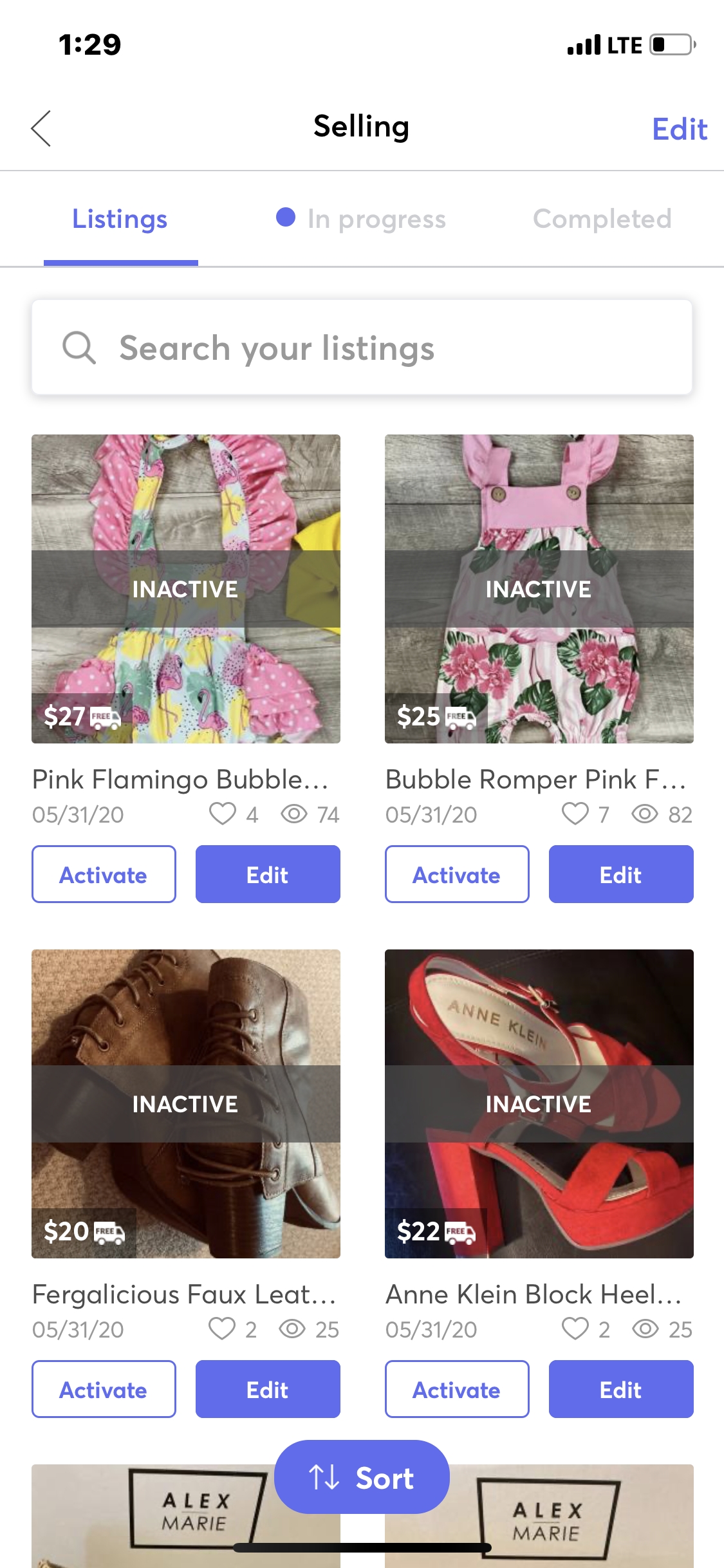This vertically rectangular screenshot from a cell phone display captures a white background interface. At the top left, the time is shown in black as "1:29," while on the top right, there is a series of icons including the signal bar, "LTE," and the battery icon. 

Centered below these indicators, the word "Selling" is prominently displayed in bold black text. Adjacent to "Selling" on the right is the option "Edit" in blue, and to the left is a back arrow. Directly beneath "Selling," there are three selectable options: "Listings," "In Progress," and "Completed." The "Listings" option is currently active, indicated by its blue color and an underline.

Further down, a search bar is present, labeled "Search Your Listings," spanning the width of the frame. Below the search bar, there are four listings, each marked with a central banner stating "Inactive." The listings are as follows from top to bottom: "Pink Flamingo Bubble," "Bubble Romper Pink," "Fergalicious Faux Leather" (which appears to be a boot), and "Ankline Block Heel." Underneath each description, there are two side-by-side buttons labeled "Activate" and "Edit."